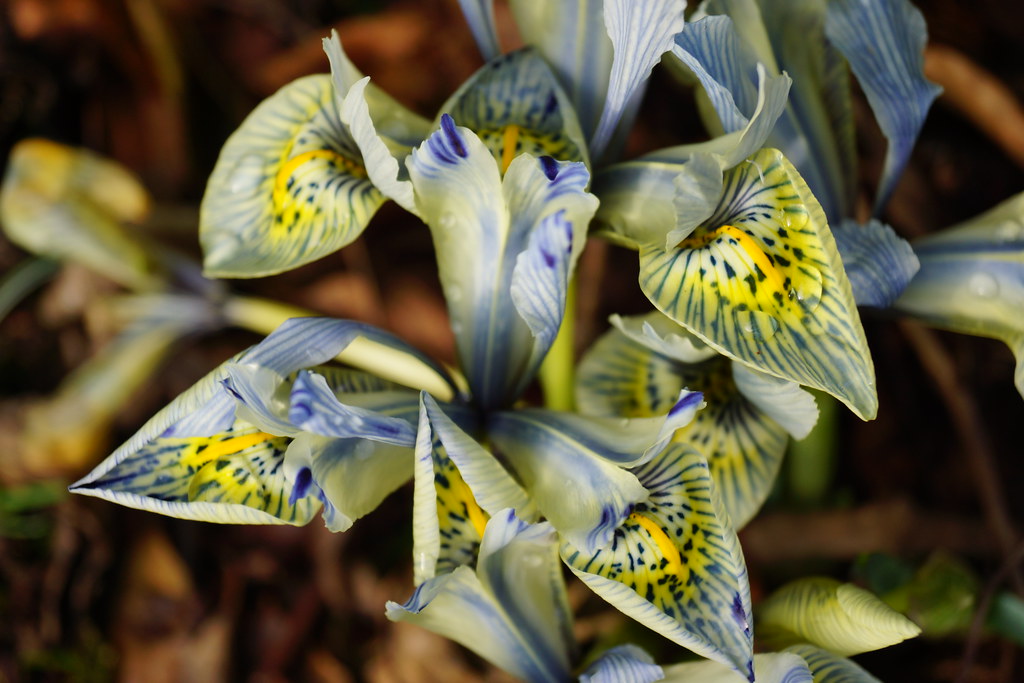This image features a close-up of approximately 5 to 10 delicate lilies, positioned at the center with a heavily blurred brownish-green background hinting at additional plants or forestry. The lily petals are a very light, almost ethereal yellow, edged with darker yellow hues and featuring intricate designs that include painted-on dark blue wispy lines, blue polka dots, and black spots. Some lilies have fine water droplets on them, adding a fresh, just-rained appearance. The centers of the lilies are bright yellow with subtle white accents, contributing to the overall vibrant texture. The blossoms, displaying both horizontal and vertical orientations, create a dynamic yet graceful composition. This beautifully intricate floral arrangement appears almost like a painted masterpiece, capturing the delicate interplay of colors and patterns on the petals.